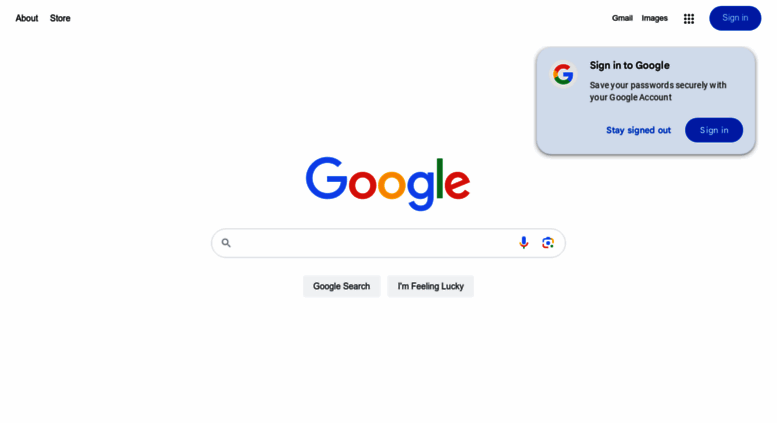The image displays a clean, uncluttered Google homepage. Dominating the center of the page is the iconic Google logo, featuring its characteristic colors: blue, red, yellow, blue, green, and red. Directly below the logo is the familiar search bar, which includes a magnifying glass icon on the left, a microphone icon on the right, and an additional icon next to it. Beneath the search bar, two clickable buttons are labeled "Google Search" and "I'm Feeling Lucky."

At the top right of the page, a notification box prompts users to "Sign in to Google," offering the option to save passwords securely with a Google account. This notification box contains two clickable options: "No thanks" in black lettering and a blue button with white text that says "Sign in."

The top left corner of the page features links labeled "About" and "Store." On the top right, there are additional links for "Gmail," "Images," and a sign-in button.

The page is minimalistic, with no other text or distracting elements, emphasizing simplicity and ease of navigation.